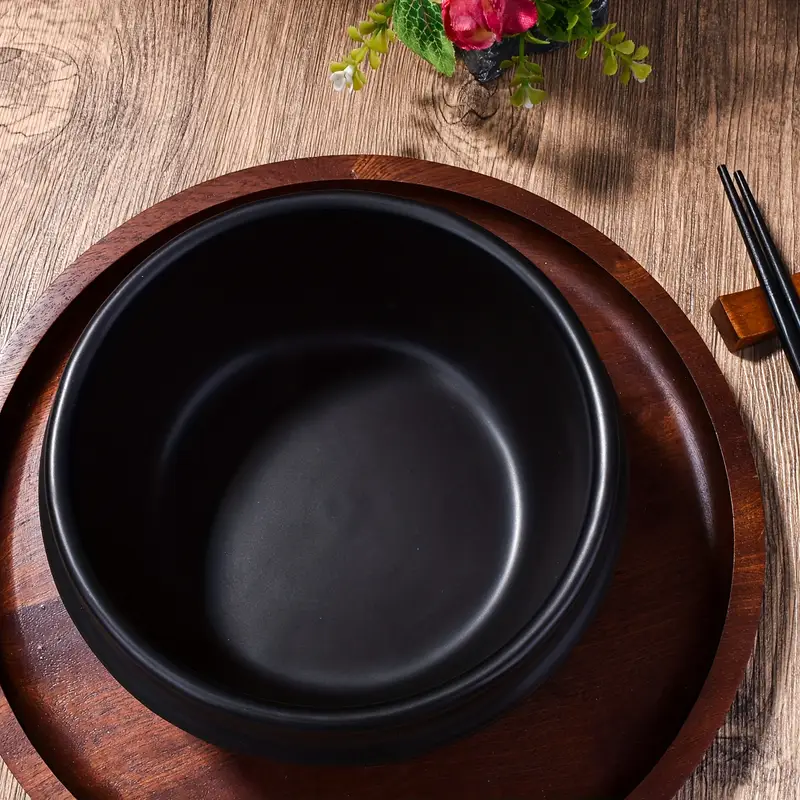The image showcases a beautifully arranged table setting. At the center, there is an empty black bowl, possibly made of plastic or pottery, resting on a dark wooden plate that has a rich grain pattern, suggesting it might be made from rosewood, cherry, or mahogany. This dark plate contrasts nicely with the light brown wooden table beneath. To the right of the bowl, a pair of chopsticks rest on a small wooden block, suggesting a meal is about to be served. At the top edge of the image, hints of a floral arrangement are visible, featuring two reddish-pink flowers accompanied by green leaves, adding a touch of natural beauty to the scene.